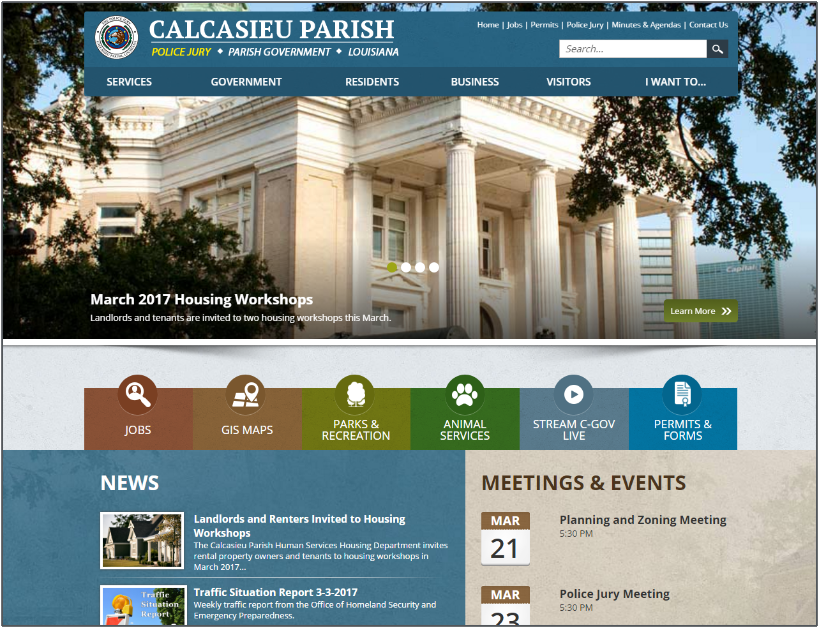This image showcases a screenshot set against a white background. The screenshot's upper half features a vivid, color photograph of a large, regal building with columns, reminiscent of an old library. At the top of the screenshot is a blue banner with the text "Calcasieu Parish Police Jury" in yellow, and "Parish Government Louisiana" in white to the right. Adjacent to this text, a white search bar is visible. Above the search bar, the menu includes options labeled "Home," "Jobs," "Permits," "Police Jury," "Minutes & Agendas," and "Contact Us." Below this in a darker blue banner, another menu displays the options "Services," "Government," "Residents," "Business," "Visitors," and "I Want To" in white text. Positioned beneath the building's image is the text "March 2017 Housing Workshops" in white.